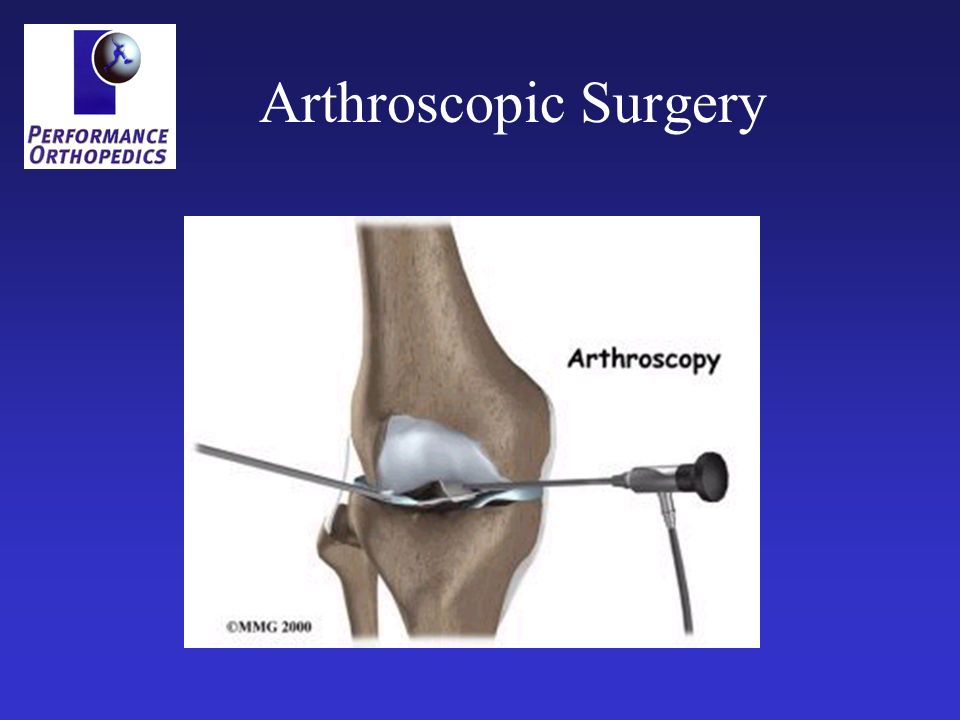The image depicts a detailed medical diagram set against a predominantly blue background. In the upper left corner, a small white rectangle displays the text "Performance Orthopedics." At the very top of the blue background, the title "Arthroscopic Surgery" is prominently featured. Central to the composition is a white square containing a detailed illustration of a joint being operated on, labeled "Arthroscopy" to the side. Two different surgical instruments are shown entering the joint from opposite sides, visibly engaging in the procedure. The bottom of the image contains the text "MMG 2000" along with a copyright symbol. The color palette includes shades of royal blue, navy blue, light blue, white, gray, black, and brown, giving it a professional and clinical appearance. The layout and style suggest that this image might serve as an informative infographic possibly designed for a medical textbook or a website related to orthopedic surgery.